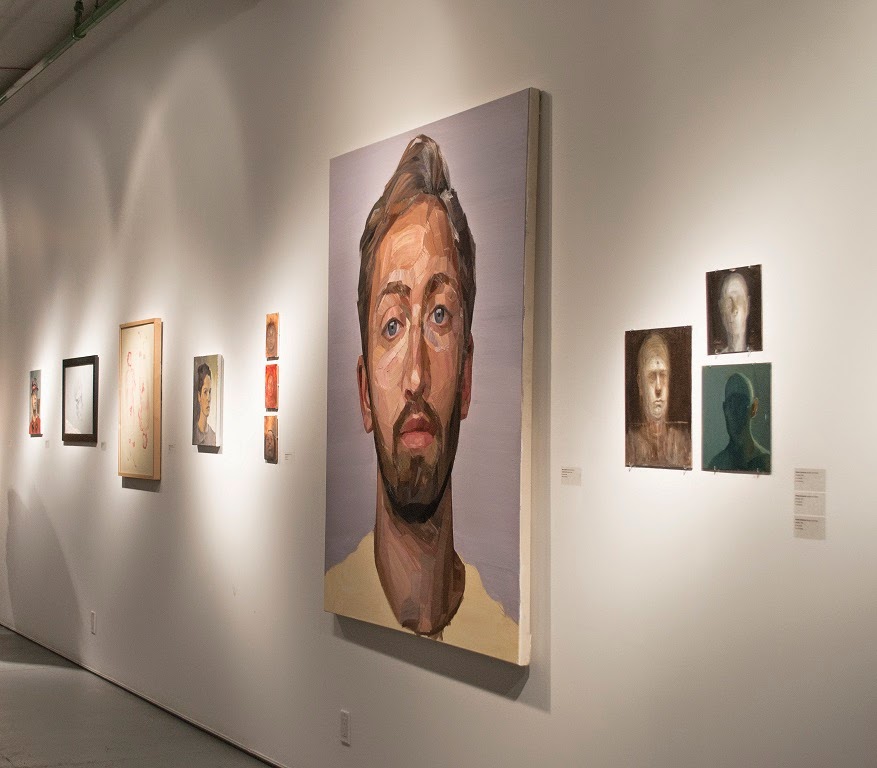This detailed caption merges information from all three captions:

Inside a whitewashed gallery in a museum, there is an art show, possibly featuring student work. A prominent feature on one of the walls is a very large, unframed canvas portrait of a man that closely resembles Hugh Laurie. The portrait is impressionistic, rendered in oil paints with a vivid array of colors to detail his dark hair, which includes shades of brown, light brown, and white highlights for depth. He has a peachy skin tone with distinct shading on his full lips and nose. His facial hair is dark, framing his blue, piercing eyes and large ears. The man, wearing a yellow t-shirt, stares directly forward with a serious expression. 

Around this main portrait, the gallery wall features a total of 11 artworks, including both paintings and photographs. Some of these images depict people with alien-like appearances, characterized by vivid green tones and indistinct facial features. Others include more recognizable human forms, like a woman whose features are only partially clear. The arrangement of these works is varied, with some smaller pictures stacked vertically. Small plaques that provide descriptions and artist information accompany each piece, though the text is too small to be legible in the image. The scene is illuminated by track lighting above, and there's a person standing within the gallery space.